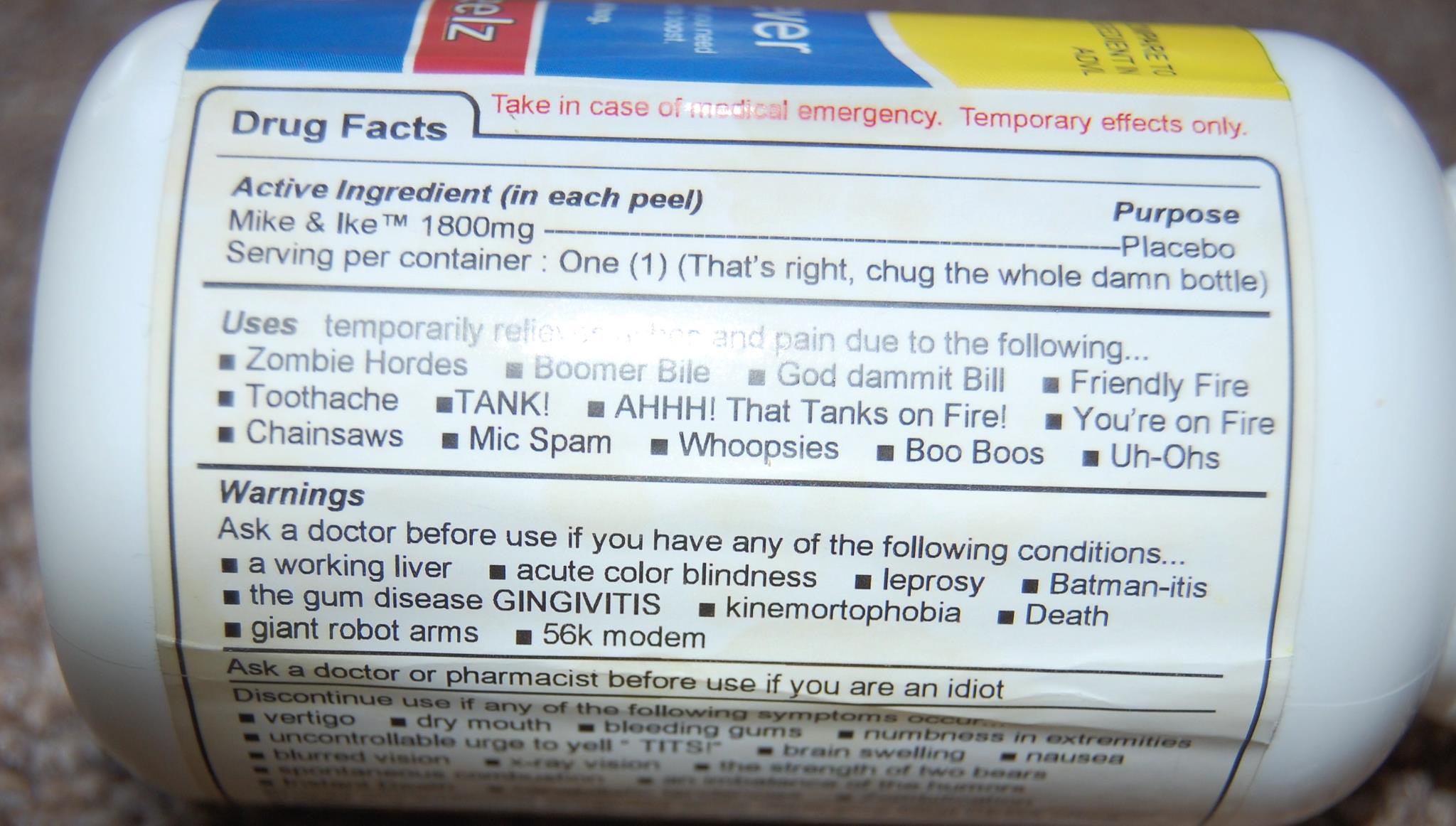A photograph captures a white plastic bottle adorned with a humorous and novelty label. The label's "Drug Facts" section lists "myconics" as the active ingredient. It humorously claims to provide temporary relief for a variety of outlandish ailments, including "zombie hordes," "goddammit Bill," "friendly fire," "toothache," "you're on fire," "chainsaws," "Mike spam," "whoopsies," "boo-boos," and "uh-ohs." The "Warnings" section advises consulting a doctor if you have conditions such as "a working liver," "acute colorblindness," "leprosy," "batman-itis," "the gum disease gingivitis," "death," "giant robot arms," or "56k modem." Additionally, it suggests asking a doctor or pharmacist before use if "you are an idiot."